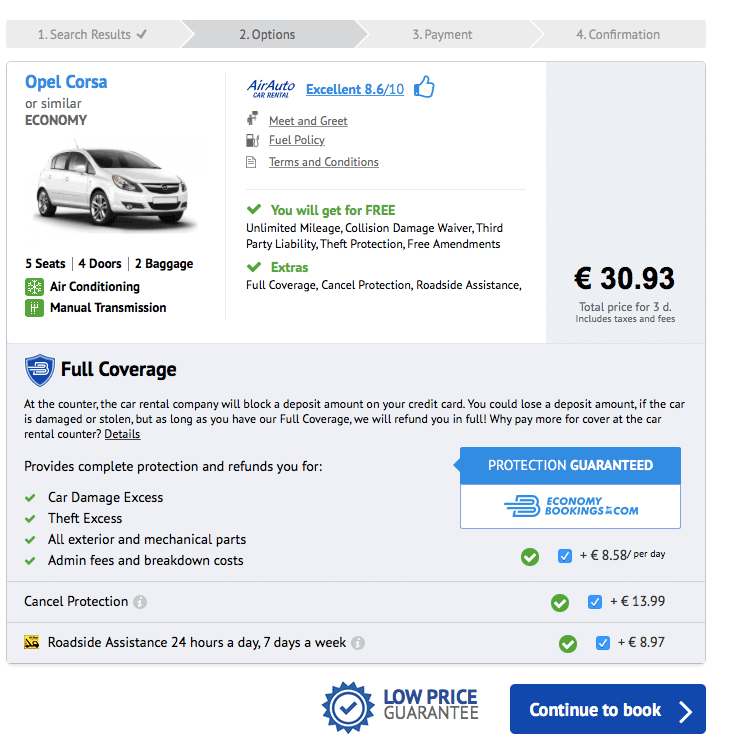This is a detailed screenshot of a car rental page from Air Auto Car Rental, displaying the charges for renting a particular vehicle. The top of the page outlines the rental process steps: Search Results, Options, Payment, and Confirmation. 

Below, the rental details for an Opel Corsa or similar economy vehicle are presented, accompanied by an image of a white car. The vehicle includes features such as free unlimited mileage, collision damage waiver, third-party liability, theft protection, and free amendments. Optional extra coverage includes full coverage, cancel protection, and roadside assistance. The car is described as having five seats, four doors, space for two pieces of baggage, air conditioning, and a manual transmission.

To the side, the total rental price for three days is shown as €30.93, inclusive of taxes and fees. Further down, a note on full coverage explains that the rental company will block a deposit amount on your credit card. In the event of the car being damaged or stolen, the deposit is at risk; however, with full coverage, the amount will be refunded in full. The section advises that opting for full coverage guarantees protection and may prevent paying additional cover fees at the rental counter. The page concludes with a blue button inviting the user to "Continue to Book."